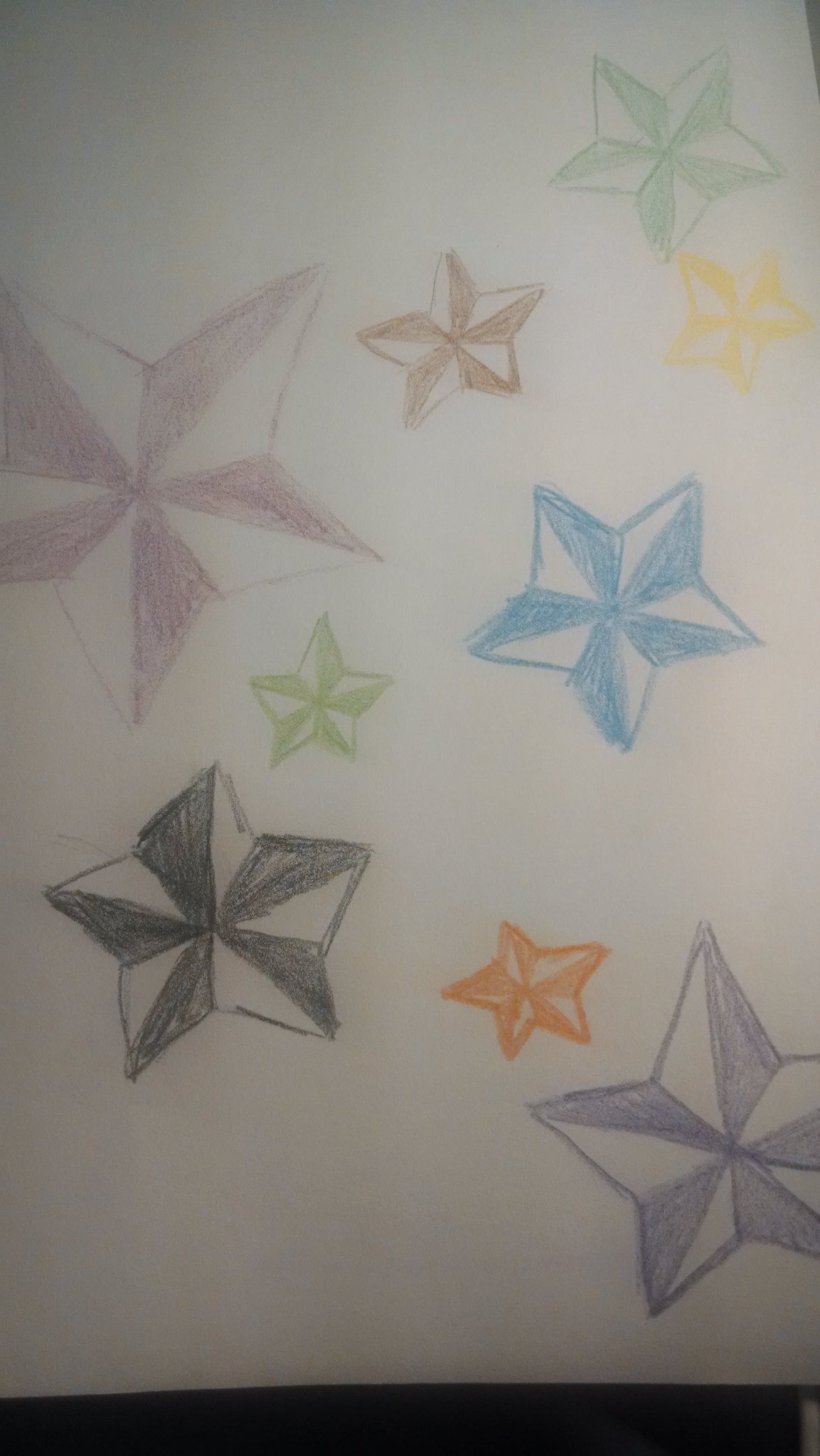This photograph features a detailed drawing of three-dimensional stars meticulously crafted on a white piece of paper. At the bottom of the image, there's a black rectangle, providing a contrasting backdrop to the vivid colors of the stars. The stars themselves are intricately outlined and colored, with each star having one half of its triangle segments filled in a distinct color that gradients towards the center, giving a 3D appearance. The stars include pairs of purple and white, orange and white, black and white, green and white, brown and white, blue and white, yellow and white, and dark red and white. They are spread across the page without any particular pattern, emphasizing their vibrant and contrasting colors. Notably, one star on the left side appears slightly larger than the others, adding a unique focal point to the otherwise seemingly random arrangement.